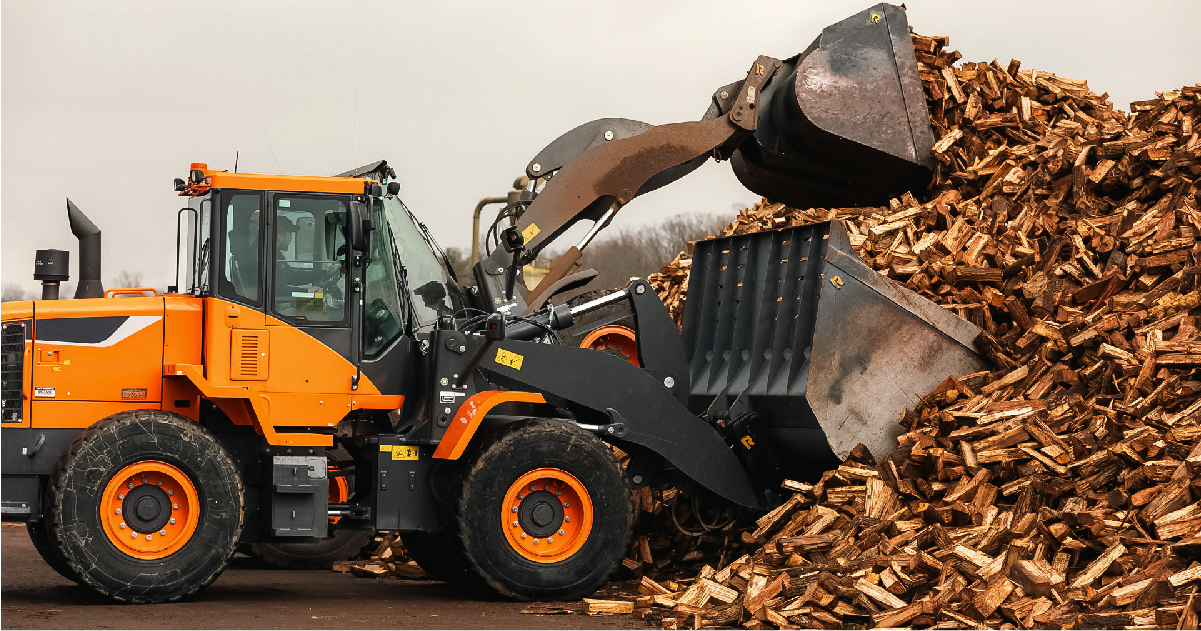The image depicts a busy worksite dominated by two large yellow excavators and a massive pile of firewood or lumber scraps. The scene is vivid with the earthy hues of browns and oranges, contrasting against a gray sky. On the left side of the image stands a pristine yellow excavator, featuring a yellow roof, black detailing on the door and engine cover, large black wheels with yellow rims, and silver bolts. Its robust structure includes black steps leading up to the cab. This excavator is equipped with two scoops: the lower scoop, hefty and steel, appears designed for pushing materials at ground level, while the upper scoop, slightly smaller, is raised and seems intended for lighter tasks. Both scoops are actively engaged in managing the sizable woodpile that spans the right-hand side of the image, towering above the machines. The excavators' diligent work ensures that piles of wood, meticulously cut for fuel or burning, are efficiently scooped and repositioned, showcasing the machinery’s powerful functionality in handling heavy-duty tasks.